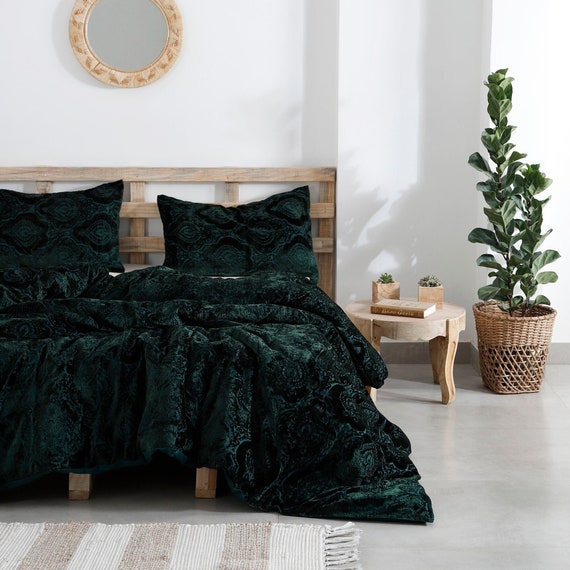This image showcases a beautifully designed bedroom with white walls and a polished concrete floor. The focal point is a bed adorned with dark jade green pillows and blankets atop a wooden frame and matching headboard, featuring vertical and horizontal slats. To the far right, a tall and vibrant fiddle leaf fern in a light brown, basket-style planter brings a touch of greenery to the room. Sitting beside the bed is a light-colored, unfinished wooden night table that holds two small wooden cube boxes containing tiny green plants and an unreadable book. At the foot of the bed lies a striped beige and white rug with fringed endings, adding texture to the space. A round mirror with a manila-colored wooden frame hangs on the wall above the headboard, reflecting the well-lit room. Shaded light casts from the right, highlighting the clean and calming ambiance of the room.